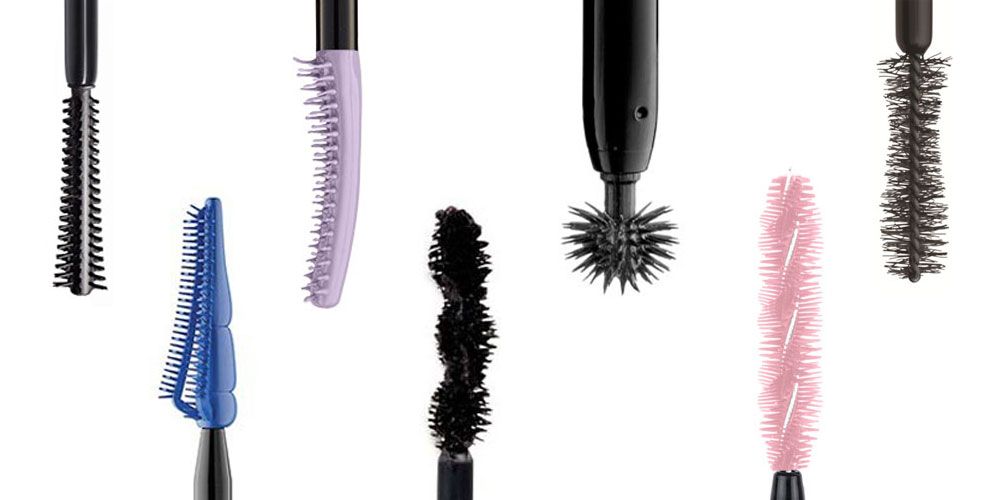The image showcases seven distinct makeup brush heads, each oriented vertically against an entirely white background. Arranged in two rows—with four on the top and three on the bottom—the brushes alternate between descending from the top edge and rising from the bottom edge of the frame. The brush heads feature various colors and designs suitable for different types of makeup application, such as eyeliner, eyebrows, or mascara.

Starting from the top left, there is an all-black cylindrical brush. Next to it is a brush with a black base and light purple bristles. Adjacent to this is a brush with a rounded head, also black. The last in the top row, on the right, is another entirely black brush. 

On the bottom row, the first brush features blue bristles and is followed by a fully black one. The final brush on the bottom right is characterized by light pink bristles. The handles of the brushes, all black, extend either down from the top of the image or up from the bottom, framing the variety of colored bristles in the center. 

Overall, this meticulous arrangement highlights the varied textures and functions of the makeup brushes, making it a comprehensive visual of tools used for detailed eye makeup applications.